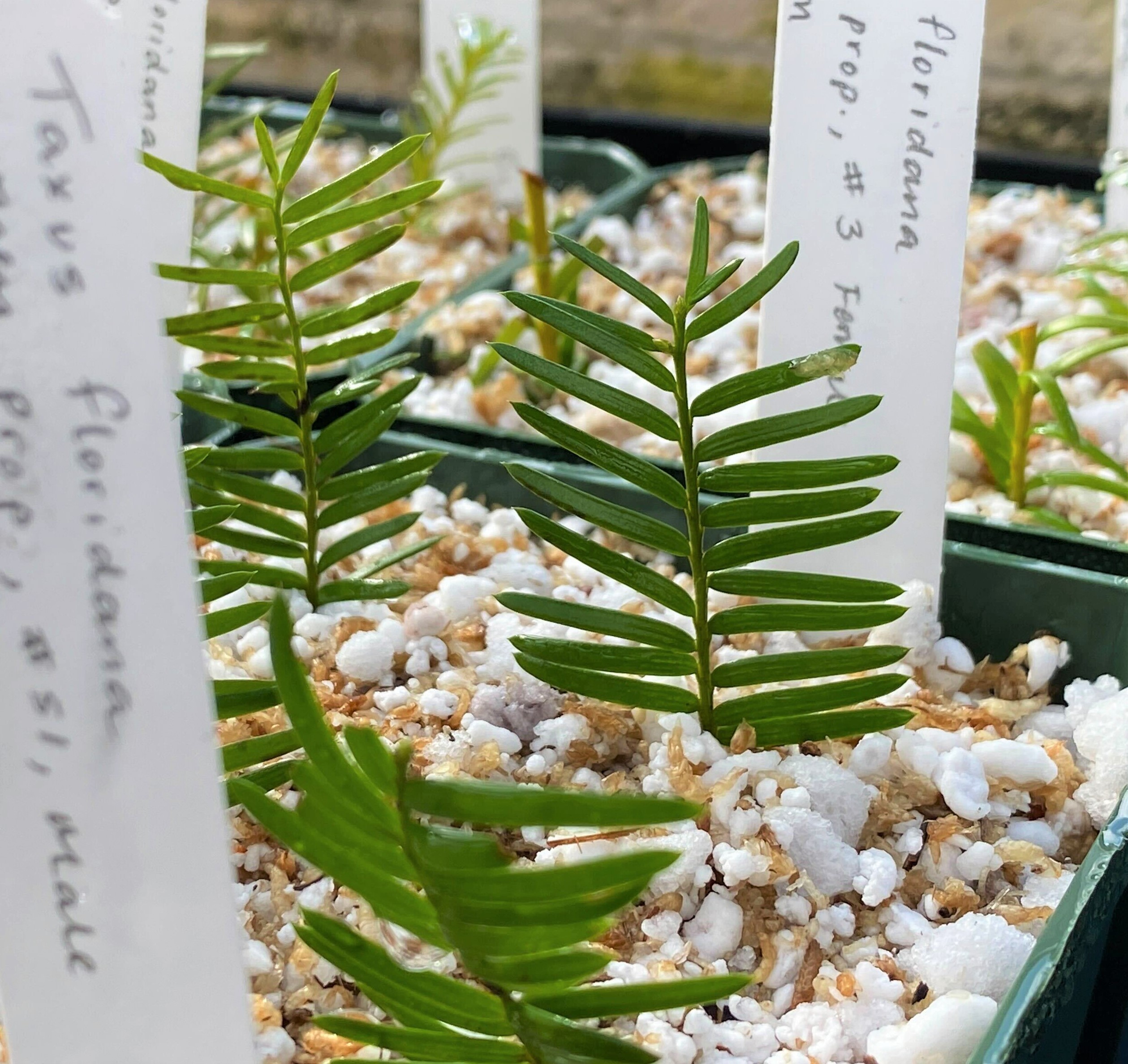The close-up square image captures three green planters, though they're partially cut off at the edges of the photograph. These planters appear to be made of ceramic or plastic and contain a mixture of white and brown particulate material, likely either a type of soil or fertilizer. Emerging from this substrate, each planter hosts four small stems with elongated, oval-shaped green leaves. Each stem is marked with a white label identifying the plant, despite the text being somewhat blurry and cut off. The labels indicate species names and details such as "Taxus floridana, number 51, male" and "Floridana, number 3, female." The planters are positioned closely together, touching one another, in what looks like a larger collection of similar containers.